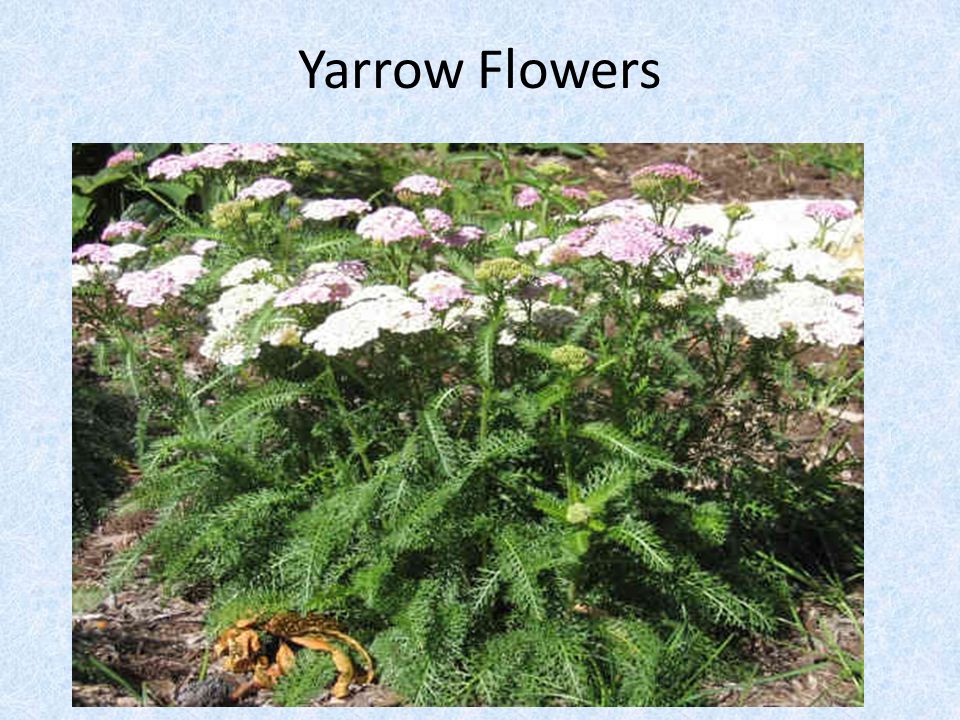This daytime photo, taken from a person's eye level, captures a lush bush adorned with numerous bright green leaves and a mix of white and lavender Yarrow flowers. The vibrant foliage fills most of the frame, with the flowers predominantly white and scattered with a few lavender blossoms, especially noticeable towards the back of the bush. The plant features green leaves resembling pine needles, adding texture to the scene. At the top of the image, text reads "Yarrow Flowers." The ground beneath the bush is primarily dirt and mulch typical of natural settings or walking trails. In the lower left corner, a brown object, possibly a dead leaf, is visible amidst the earthy backdrop, though its exact nature is unclear. The detailed composition highlights the serene beauty of the natural floral display.